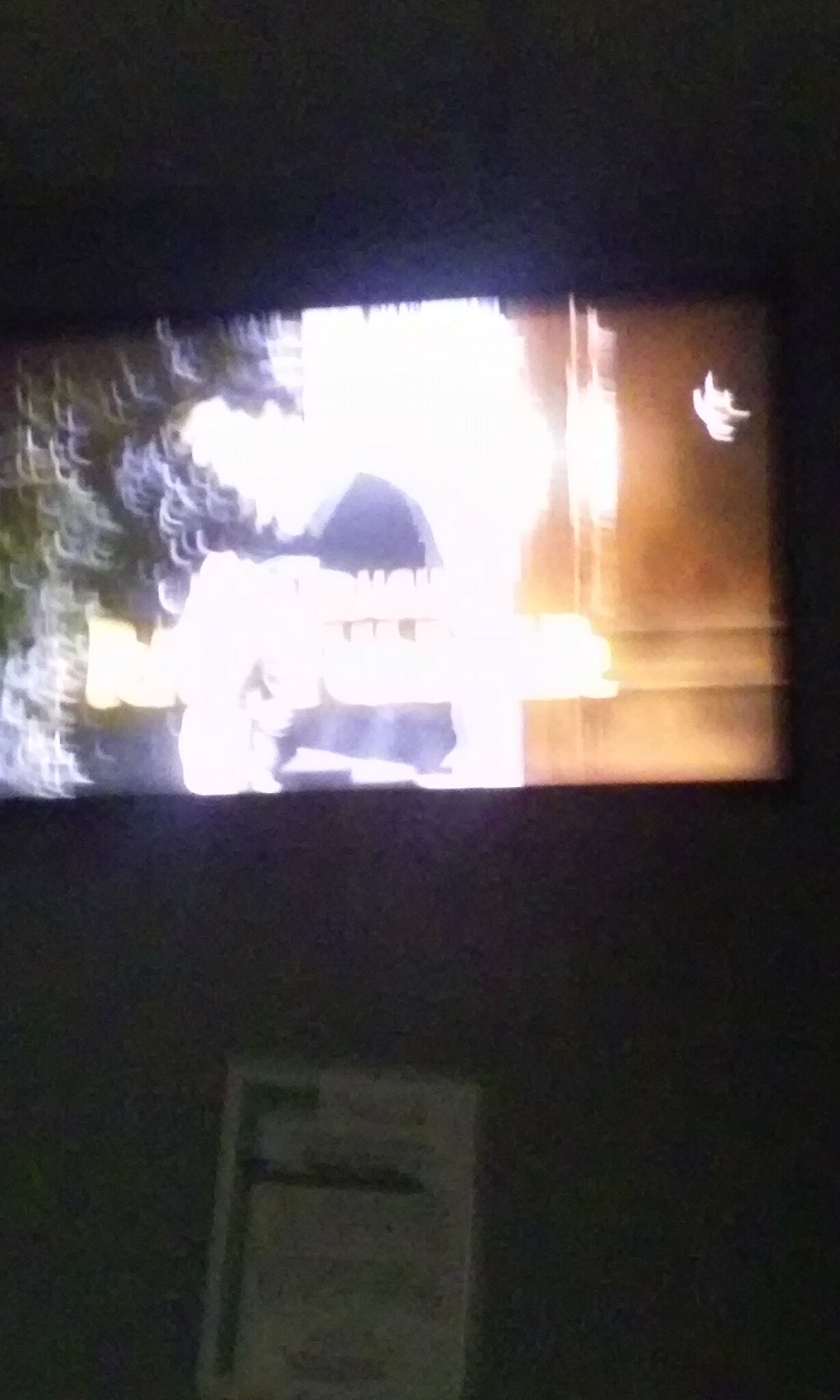This is an unclear and blurry photograph, likely taken at night. The image is dominated by darkness, with a slight green hue cast by the light from a television. The television screen itself displays a mixture of white, black, brown, and green colors, but it is overexposed, making the details indistinguishable. In the lower part of the photo, there is a white rectangular object that resembles a notebook or a sheet of paper, hanging on something. This paper shows indistinct markings and carries a green tint along with a black line, possibly forming an F-shape, though the poor quality of the image makes it hard to confirm. The overall view seems to be skewed, adding to the difficulty in discerning the exact contents and spatial arrangement within the photo.